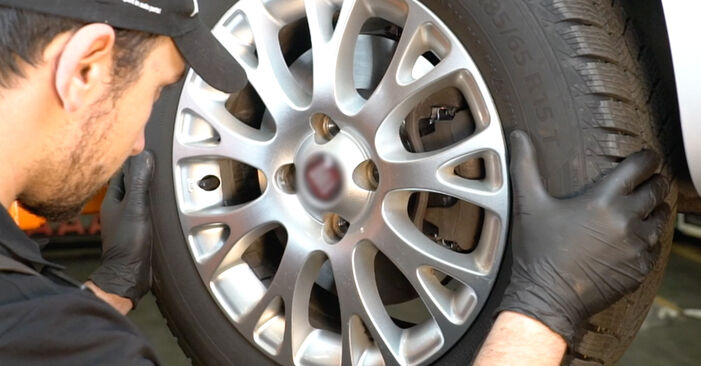A focused image captures a man attentively inspecting a tire, likely in the process of fixing it. He is positioned in the upper left corner, wearing a baseball cap that sits atop his darker black hair. His light skin and facial features, including his right ear, right eye, sideburns, and beard, are clearly visible, while his left ear and eye remain hidden from view. Dressed in a black shirt, the man’s left hand is gripping the left side of the tire, clad in a black vinyl glove that matches the one on his partially visible right wrist. The tire, prominently displayed with the marking "85-65 RTS" on the upper right corner, appears brand new and is complemented by a shiny silver rim. The rim's numerous openings reveal glimpses of the tire's internal workings. The scene's background, particularly noticeable in the bottom right corner, features slate flooring, suggesting the indoor setting of the workspace.